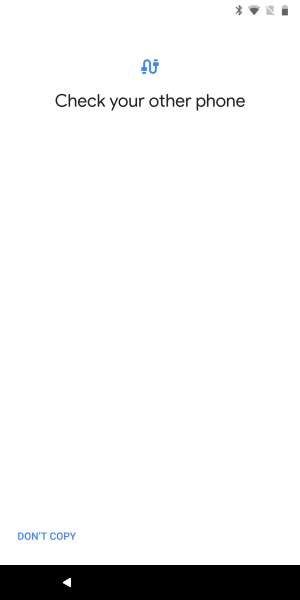A detailed screenshot of a smartphone display. In the upper right corner, there are four dark gray icons: a wireless connection symbol, an internet connection indicator showing two-thirds full, a rectangle with a line through it, and a battery icon also two-thirds full. Each of these icons has light gray highlights, with more pronounced light gray areas on the internet and battery symbols.

At the top center of the screen, a blue icon resembling an S-shaped wire with plug-ins at both ends is displayed. Under this icon, "check your other phone" is written in black text.

Towards the bottom, in bold blue capital letters, the words "DO NOT COPY" are prominently visible. The bottom of the screenshot features a black bar, containing a white triangle pointing to the left.